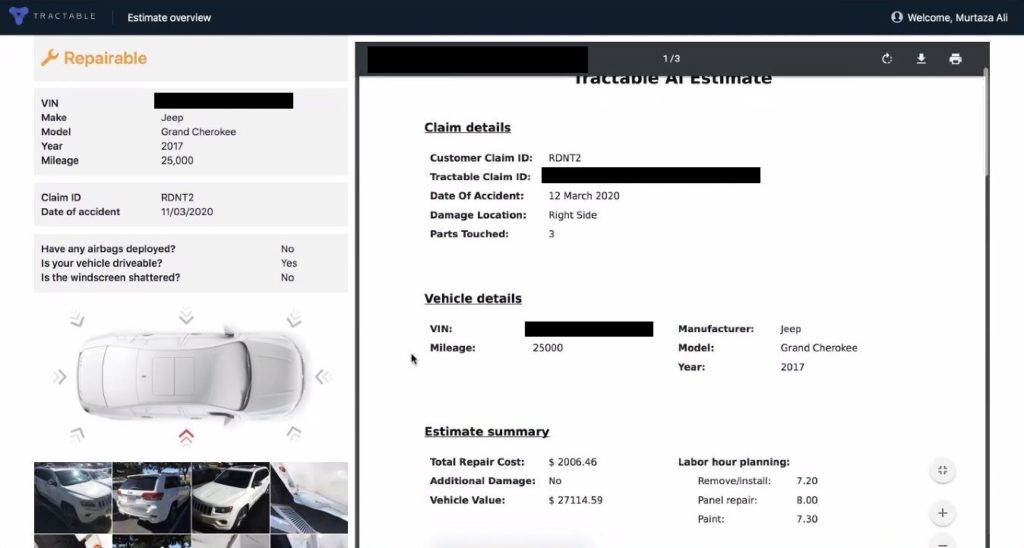The image is a detailed screenshot of a website featuring a specific vehicle accident claim overview.

At the top of the screenshot is a black bar featuring a blue logo and the word "Tractable." To the right, there is a section labeled "Estimate Overview." Further right, a profile icon appears with the caption, "Welcome, Murtaza Ali."

Beneath this section are two primary columns:

- **Left Column:**
    - A wrench icon with the label "Repairable."
    - Vehicle Information:
        - **VIN:** [Blacked out]
        - **Make:** Jeep
        - **Model:** Grand Cherokee
        - **Year:** 2017
        - **Mileage:** 25,000 miles
        - **Claim ID:** RDNT2
        - **Date of Accident:** 11-3-2020
        - **Airbags Deployed:** No
        - **Is the Vehicle Drivable:** Yes
        - **Windscreen Shattered:** No
    
    - Below this information is an aerial view image of the vehicle indicating damage points:
        - All arrows are grey except a red arrow pointing to damage near the passenger side door.
        
    - Four thumbnail images of what appears to be a white SUV, presumably showing the vehicle's damage; however, the thumbnails are too small to discern details clearly.

- **Middle and Right Columns:**
    - A black bar at the top with "1 of 3," accompanied by refresh, download, and printer symbols.

    - A partially readable heading ending with the word "Estimate".
    
    - Claim Details:
        - **Customer Claim ID:** RDNT2
        - **Tractable Claim ID:** [Blacked out]
        - **Date of Accident:** 12 March 2020
        - **Damage Location:** Right side
        - **Parts Touched:** 3
    
    - Vehicle Details:
        - **Manufacturer:** Jeep
        - **Mileage:** 25,000
        - **Model:** Grand Cherokee
        - **Year:** 2017
    
    - Accident Summary:
        - **Total Repair Cost:** $2,006.46
        - **Additional Damage:** No
        - **Vehicle Value:** $27,114.59
    
    - Labor Hour Planning:
        - **Remove/Install:** 7.20 hours
        - **Panel Repair:** 8.00 hours
        - **Paint:** 7.30 hours
        
    - At the bottom right are symbols, including a plus and minus sign, and an unidentified symbol.